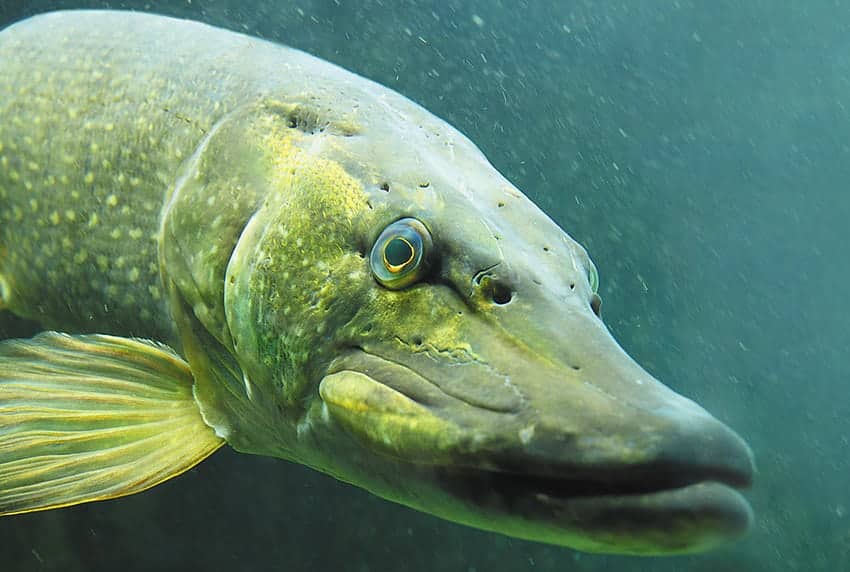This is a detailed close-up photograph of a catfish taken underwater. The fish is angled at approximately 45 degrees toward the camera, allowing only its right eye— which appears quite metallic and piercing—to be visible. Its body is predominantly green with yellowish hues, especially around the midsection where yellow dots are noticeable. The fin is more yellowish, while the top part of its head near the mouth is a darker green. There are holes at the top of its head, suggesting they are used for breathing. The background is a teal blue water filled with small whitish particles, creating a serene aquatic environment. The fish seems to be in motion, possibly performing a maneuver, and the photo appears to be taken during the daytime.